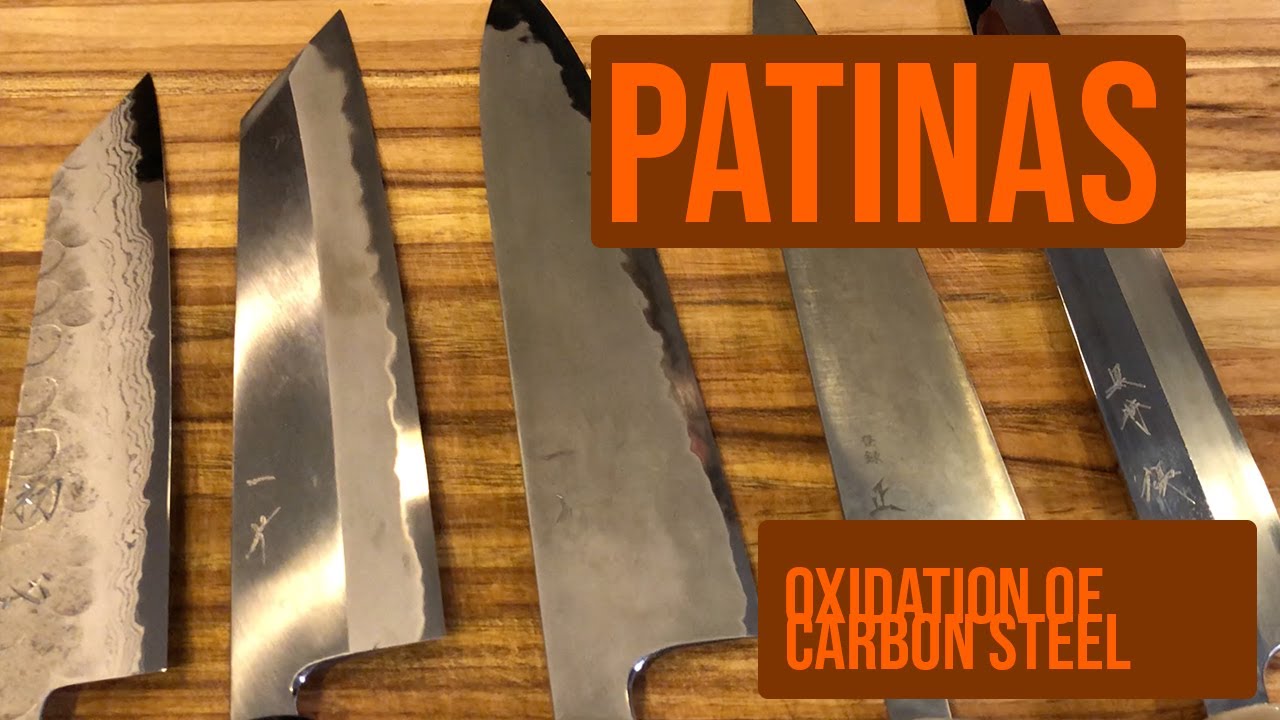The photograph showcases five distinct knives of varying shapes and sizes, all aligned with their blades facing right on a richly grained wooden cutting board. Each knife, characterized by different shades of silver, exhibits signs of extensive use and wear, highlighting their well-worn edges and unique patinas. This suggests a history of diligent utilization, hinting at their role in professional culinary settings. Overlaid on the image, the word "PATINAS" is prominently displayed in large orange letters against a darker brown background. Beneath it, the phrase "oxidation of carbon steel" is presented in a smaller orange font. The composition of the photograph, combined with the text, suggests an emphasis on the natural aging process of carbon steel knives, likely serving as an advertisement or educational piece about the effects of oxidation on metal tools.